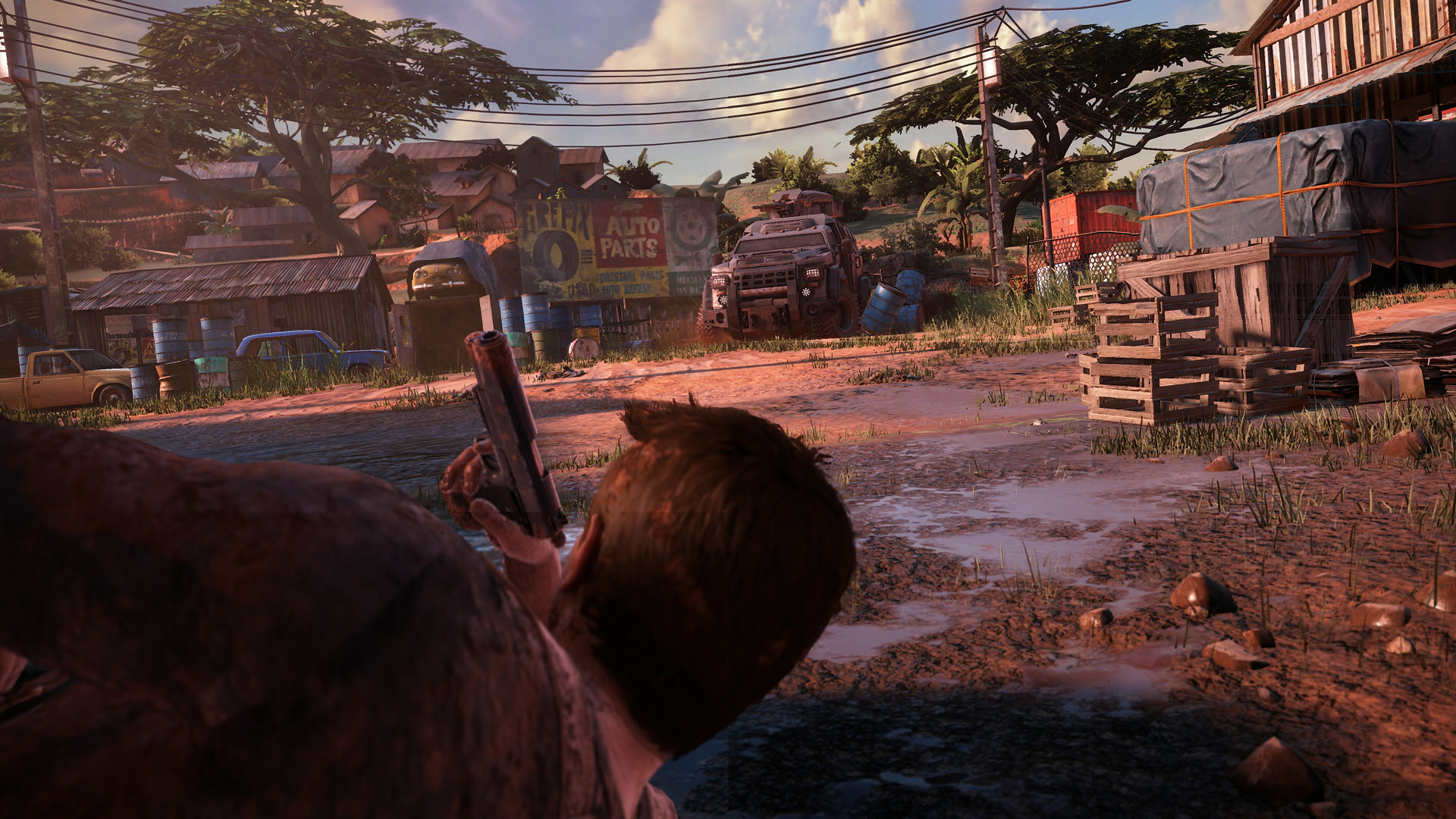In the detailed screen capture of an action video game scene, the focus is on a man with brown hair and a dark brown jacket or coat, lying on his right side behind a barrel or pipe, in a parking turnaround area scattered with rocks and mud puddles. He clutches a pistol in his right hand, appearing to conceal himself cautiously. The setting features an outdoor scene dominated by an aluminum or metal warehouse with a large open dock, surrounded by stacked wooden crates and a massive bulk pack wrapped in black plastic with red strapping. Across the street from the warehouse, there is a rundown auto parts store with a sign reading "Auto Parts" in white letters against a red background, featuring a tire logo. Vehicles are parked in front of the store, including an orange pickup truck, a blue car, and a large, possibly junked heavy equipment truck. Additional elements include a railroad track, various trees, power lines running through the scene, and a clear blue sky dotted with white, puffy cumulus clouds.